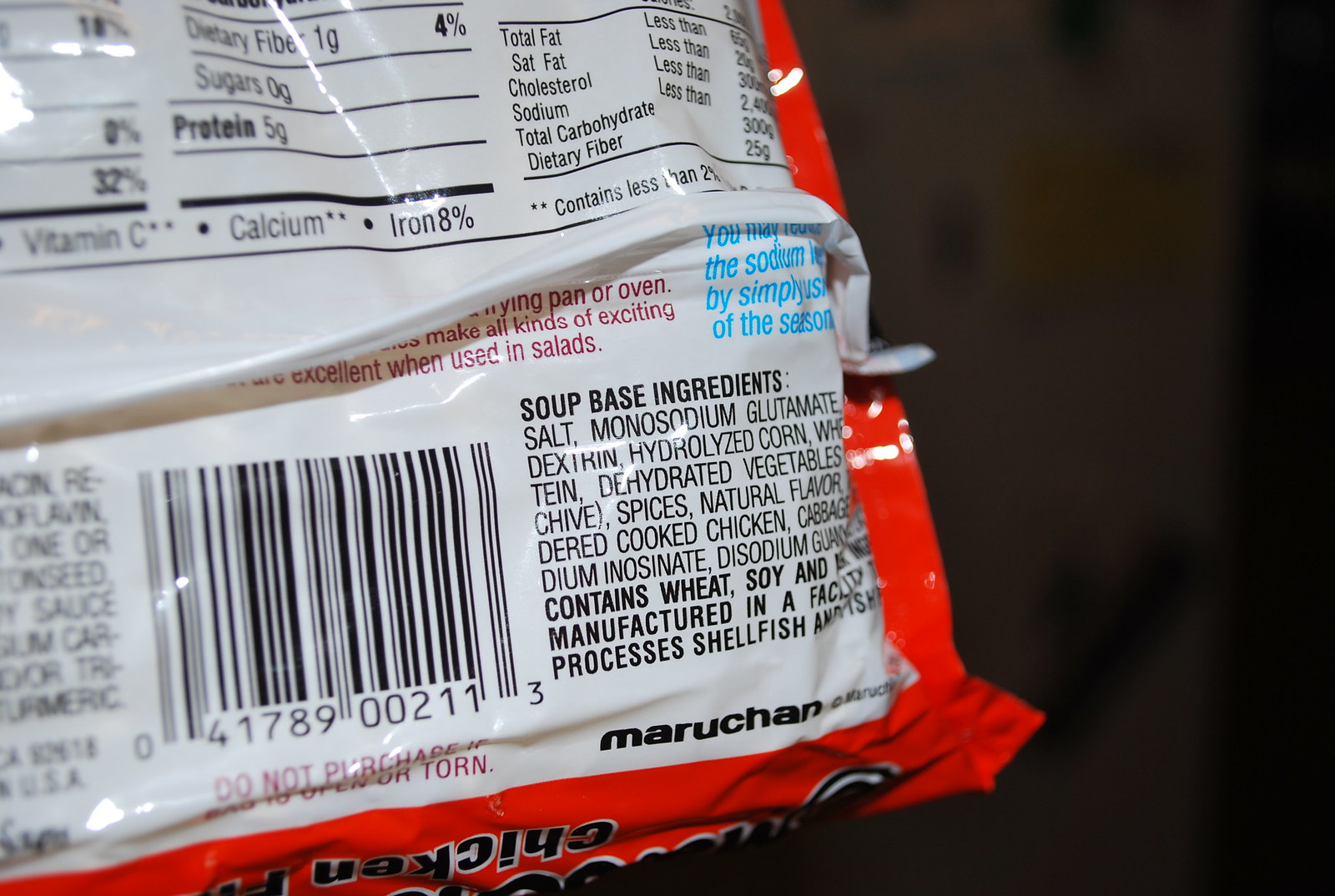The image showcases a Maruchan chicken-flavor ramen noodle package against a black background. On the left side of the package, the word "bag" is clearly visible against the dark backdrop. There is a prominently displayed warning advising not to purchase the product if the packaging is torn, located at the bottom right corner. The bottom-right corner also prominently features the Maruchan logo and the word "chicken" in bold lettering.

The package has a combination of red and white folds, with a noticeable white fold running through the middle. The top part of the package provides nutritional information, detailing dietary fiber and protein content with values of 70 grams for dietary fiber and 5 grams for protein, along with calcium at 18%. It also lists total fat, saturated fat, cholesterol, sodium, total fiber, and dietary fiber, among other nutritional facts.

Centered on the package, there are barcodes reading "5179 002 001," surrounded by additional nutritional and ingredient information. The ingredients list includes soup base components such as salt, gluten, sodium glutamate, dextrin, hydrochloride, mineralized corn, dehydrated vegetables like chives, various spices, natural flavoring, and cooked chicken. The packaging also mentions that it contains wheat and soy, and is manufactured in a facility that processes shellfish.